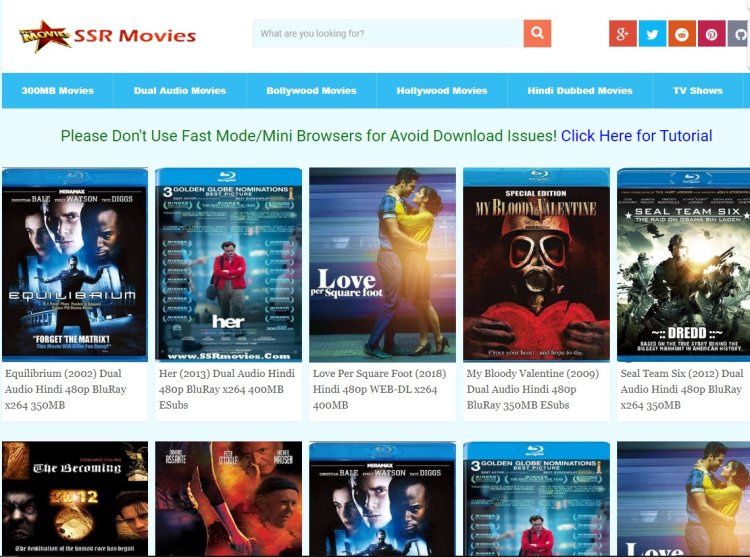The image depicts a website interface for streaming or downloading movies, titled "SSR Movies." The title "SSR Movies" is prominently displayed in red, accompanied by a stylized red star with a gold border. A search bar on the right prompts the user with the question, "What are you looking for?" 

On the far right, there are icons for various social media platforms, including Google+, Twitter, Reddit, Pinterest, and an unidentified gray icon, providing users with options to follow SSR Movies on those social networks. 

Below the social media icons, a set of blue navigation tabs offer categories such as "300 MB Movies" (indicating smaller file size movies), "Dual Audio Movies," "Bollywood Movies," "Hollywood Movies," "Hindi Dub Movies," and "TV Shows." There is also a blue link labeled "Click here for tutorial."

The main content area showcases a grid of movie thumbnails, with five movies per row and a total of ten featured movies. Each thumbnail includes the movie's title, release year, available audio options, and video quality. The first row features "Equilibrium" (2002, dual audio, 480p Blu-ray), "Her," "Love Per Square Foot," "My Bloody Valentine," and "SEAL Team 6." Each thumbnail displays the blu-ray or DVD case, allowing users to see the cover art and actors.

The second row includes titles like "The Becoming." However, one of the movies in this row is missing a title, and the last three entries are "Mystique," "Her," and another "Love Per Square Foot," repeating twice in the listing.